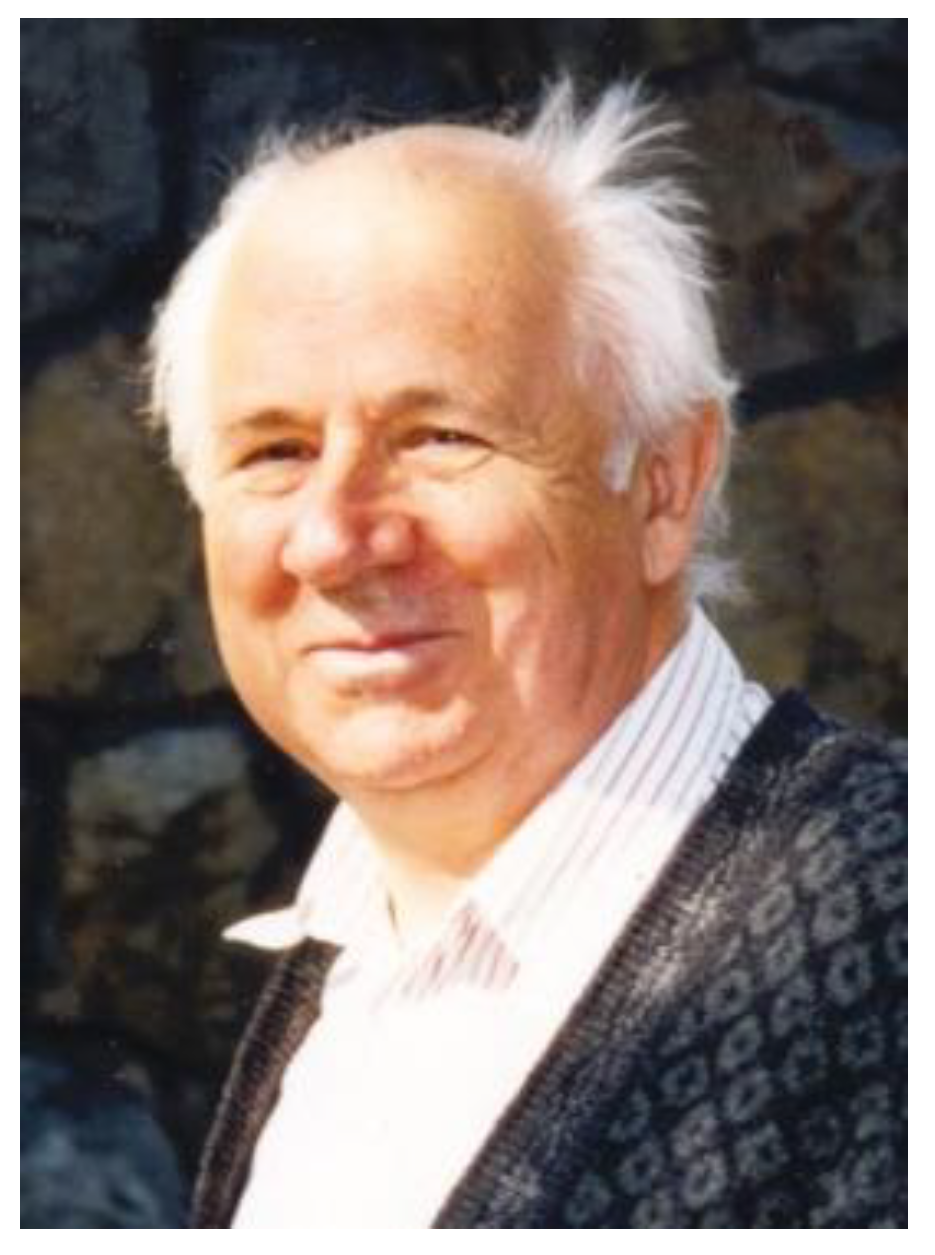The image is a grainy, blurry photograph from what appears to be the 1970s or 1980s, characterized by its low quality. It features an older man positioned in front of a rock wall composed of large, dark gray and brown stones. This man is bald on top with white hair on the sides that appears to be blowing in the wind. He has a tan complexion and a prominent nose. Dressed in a white, striped button-up shirt with a black sweater featuring white circle or diamond-shaped patterns, he strikes a pose slightly turned to the side. His expression is a smirk, with squinting eyes possibly due to sunlight illuminating his face, giving the photograph a sunny day atmosphere. The man's head and chest are the focus, resembling an old-fashioned headshot or business portrait.